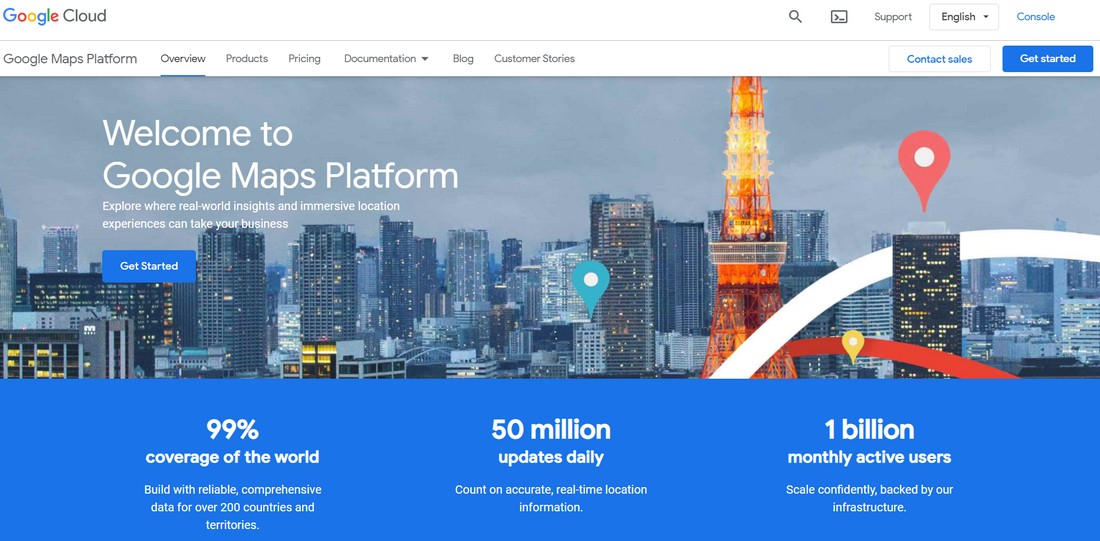The image showcases the Google Cloud website, specifically the Google Maps Platform page. The top left corner prominently displays the Google Cloud logo, with "Google" written in its unique colorful scheme of blue, red, yellow, blue, green, and red. The website header is white, featuring essential icons such as a search bar, support, language options (English), and an option named "Control" highlighted in blue.

Beneath the header, a navigation bar contains tabs including Google Map, Platform, Overview, Product, Pricing, Documentation, Blog, and Customer Stories. The currently selected tab is "Overview," indicated by a blue underline. On the top right, two buttons are visible: "Contact Sales" in white and "Get Started" in blue.

Dominating the central part of the page, the headline reads "Welcome to Google Maps Platform," followed by a subheading that invites users to "Explore where real-world insights and immersive location experiences can take your business." Below this text, there is a blue "Get Started" button.

An image of the Eiffel Tower, illuminated in yellow and brown hues, is positioned centrally, with buildings and colorful location pins (green, red, and yellow) in the background. The lower portion of the image has a blue background with white text detailing key statistics: "99% coverage of the world, built with reliable, comprehensive data for over 200 countries and territories, 50 million updates daily, count on accurate real-time location information, 1 billion monthly active users, scale confidently, backed by your infrastructure."